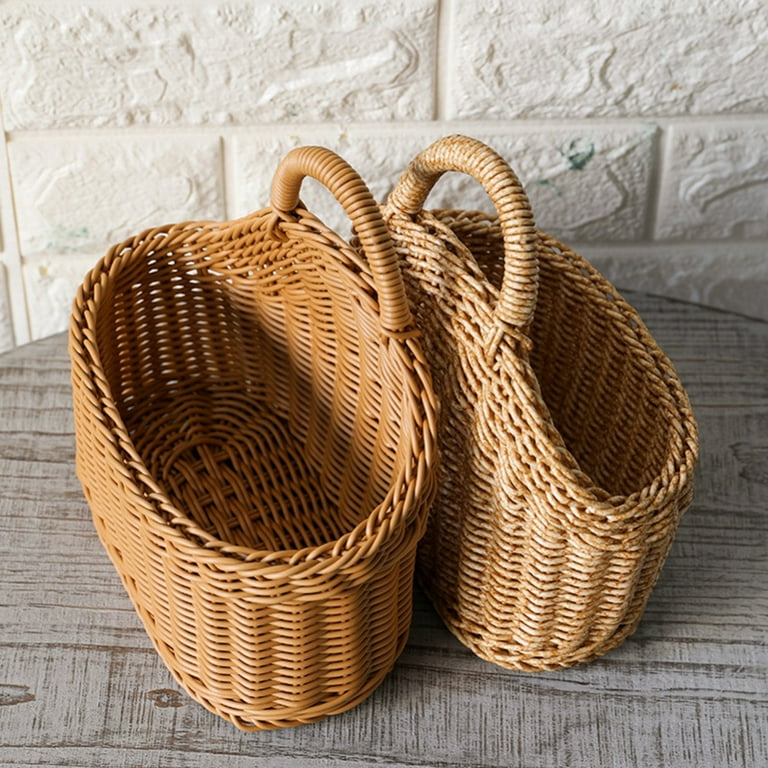This is a detailed photograph showing two empty, woven wicker baskets on a light gray flat surface, possibly a tabletop. The baskets, which seem to be handmade, have intricate designs and are various shades of brown, with one being slightly lighter and wider than the other. The handles of the baskets are positioned back-to-back at the center of the image. Behind the baskets, there's a cream-colored brick wall with noticeable greenish stains scattered across the surface. The background bricks are rectangular and contribute a stone-like texture to the setting.